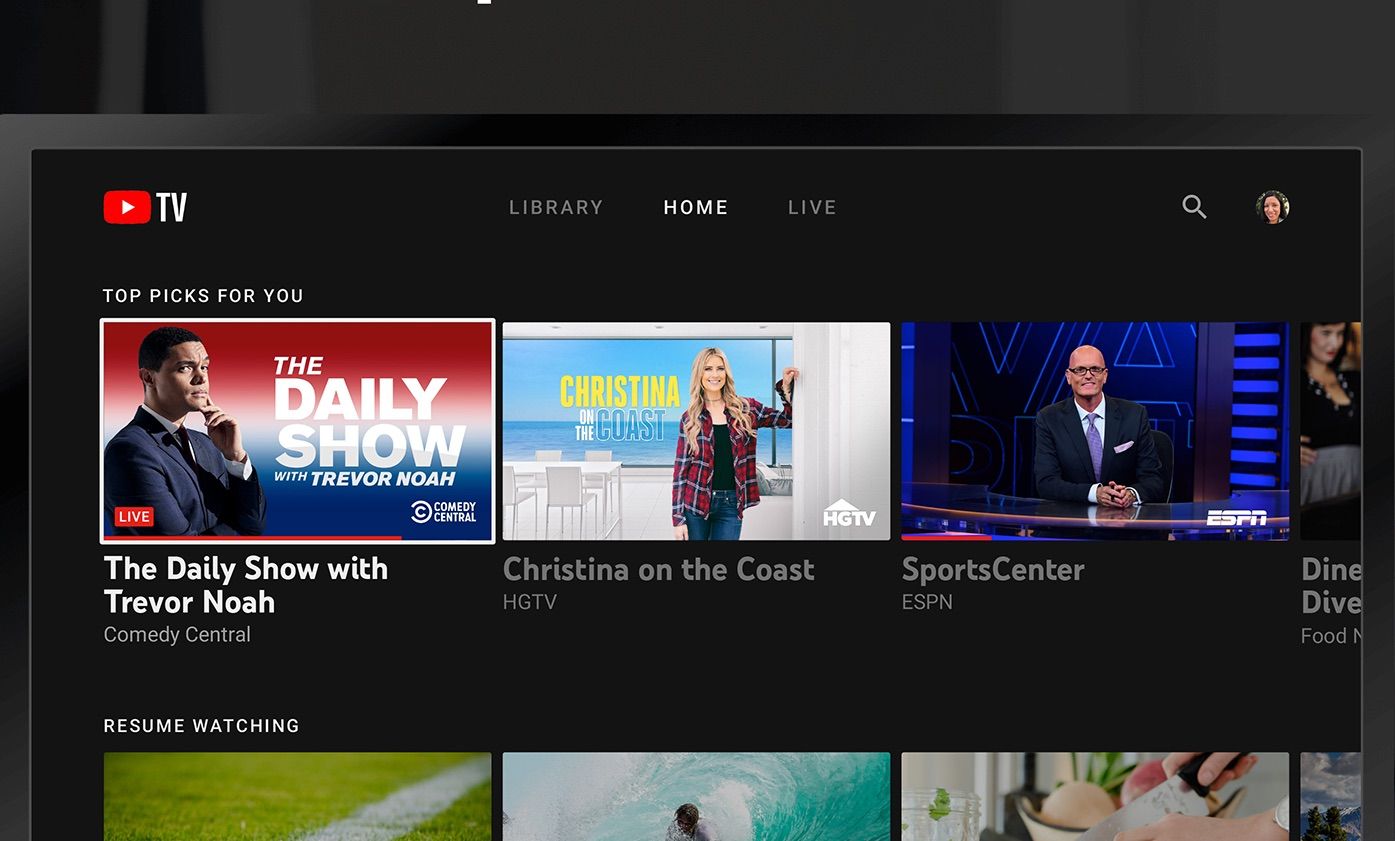This image showcases the YouTube TV home screen against a black background. In the top left corner, the iconic YouTube logo features a red play button with a white triangle, followed by the word “TV” indicating the platform YouTube TV. As we move to the right, several navigation tabs are displayed: Library, Home, and Live. These tabs are written in grey, except for the Home tab which is highlighted in white, indicating the current selection.

On the top right, a grey search icon is visible next to the user profile picture, which features an image of a woman. Below the navigation tabs, the section titled "Top Picks for You" is displayed, as this falls under the “Home” category.

The first recommendation is "The Daily Show with Trevor Noah" from Comedy Central, featuring an image of Trevor Noah in a navy suit. The show's title is split, with the top half appearing in red and the bottom half in blue.

The second recommendation is "Christina on the Coast" from HGTV, set against a backdrop of a blue river, sea, or ocean, highlighting Christina in the foreground.

To the right, "SportsCenter" from ESPN is showcased, featuring an individual in a black suit, white shirt, and purple tie seated at a table. The background is a mix of blue and dark blue hues.

At the bottom, there is a section labeled "Resume Watching," though the images for these selections are currently placeholders indicating the option to cast the content.